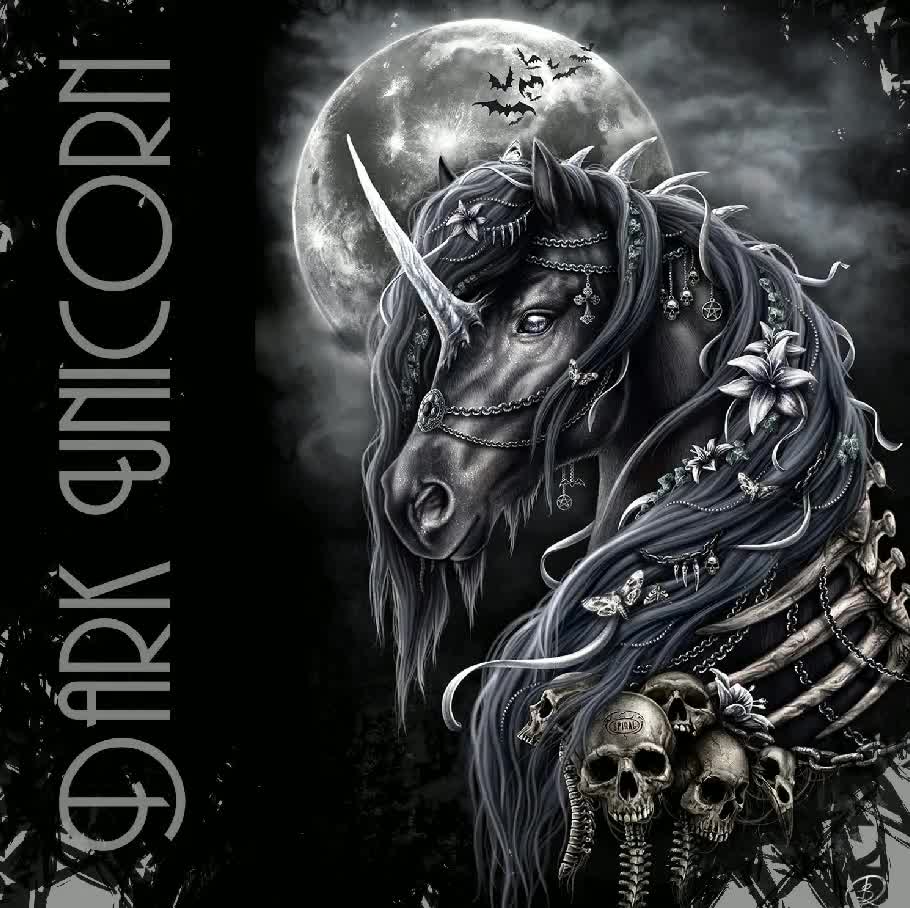This detailed black-and-white fantasy poster depicts a dark, computer-generated unicorn. The unicorn, rendered in white with sinister glassy, almost snake-like eyes, stands vertically against a full moon backdrop, creating a dramatic night scene. Adorned with elaborate jewelry, including chains across its nose and forehead, and a prominent medallion, it exudes an eerie elegance. Dark flowers entwine its mane, and scattered across its form are macabre elements like skulls, spines, and bones, enhancing its haunting appearance. Flying bats silhouetted against the moon add to the ominous ambiance. Titled "Dark Unicorn," this midnight setting captures a Halloween-like, spooky atmosphere, emphasizing the unicorn’s menacing and otherworldly allure.